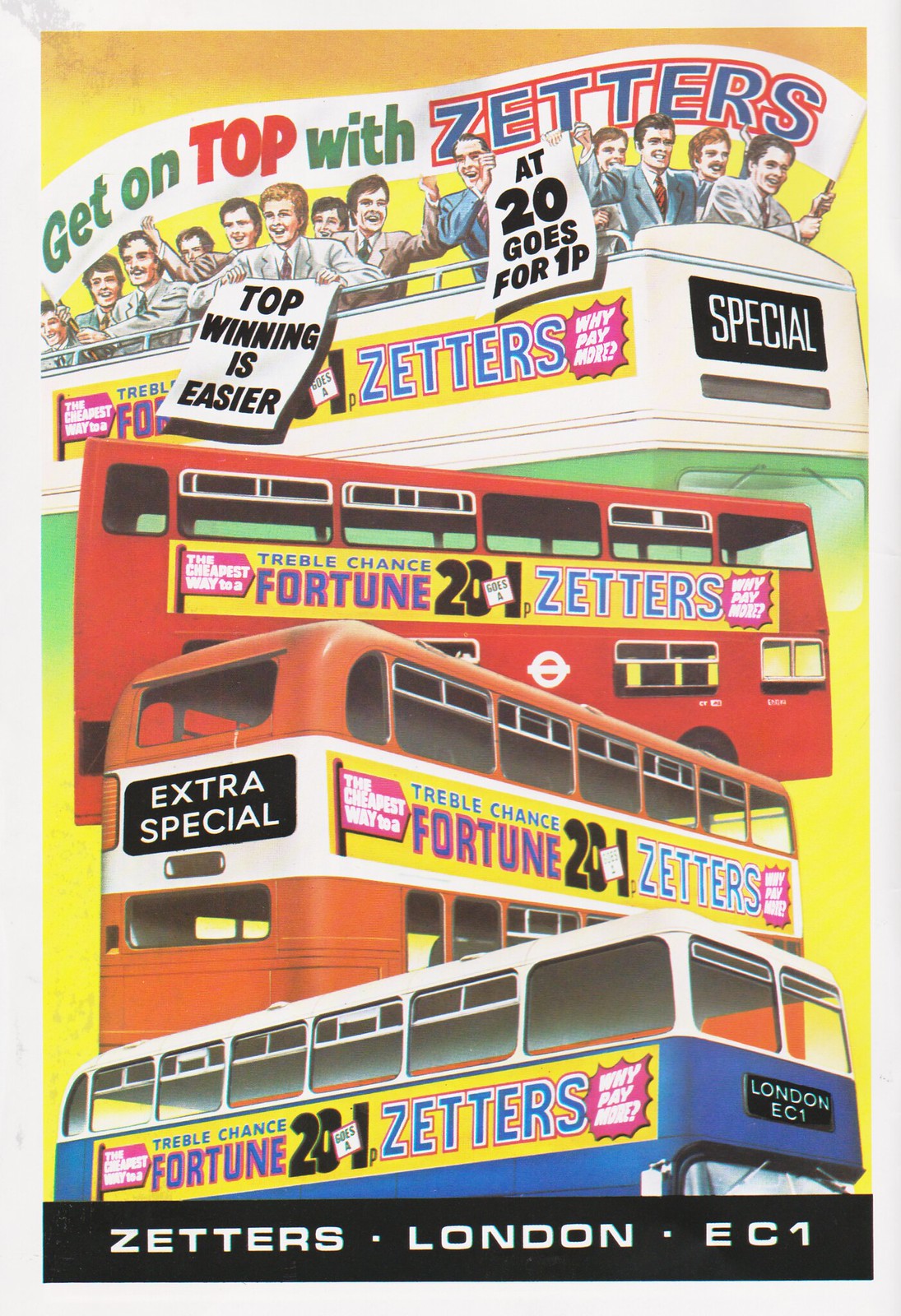This vintage flyer from the 1960s-1970s advertises for Zetters and features an eye-catching design. Dominated by stacked double-deck buses in white, red, orange, and blue, the flyer showcases a colorful and vibrant display. At the top, within a white banner, the prominent text reads "Get on Top with Zetters," emphasizing the ease of winning: "Top winning is easier at 20 goes for 1p special." The buses are not just vehicles but form part of a lively scene with cartoon drawings of men in various colored suits (gray, blue) holding a sign that reiterates "Top winning is easier." Key offers such as "extra special," "treble chance fortune 21," and "why pay more" are highlighted throughout the poster. The background features a gold, greenish-yellow color, adding depth and contrast to the white edges of the rectangular shape. Each bus sports a yellow banner with catchy phrases in vibrant colors, drawing attention to the deals Zetters has to offer. The flyer concludes with a black bar at the bottom, clearly stating "Zetters, London EC1."